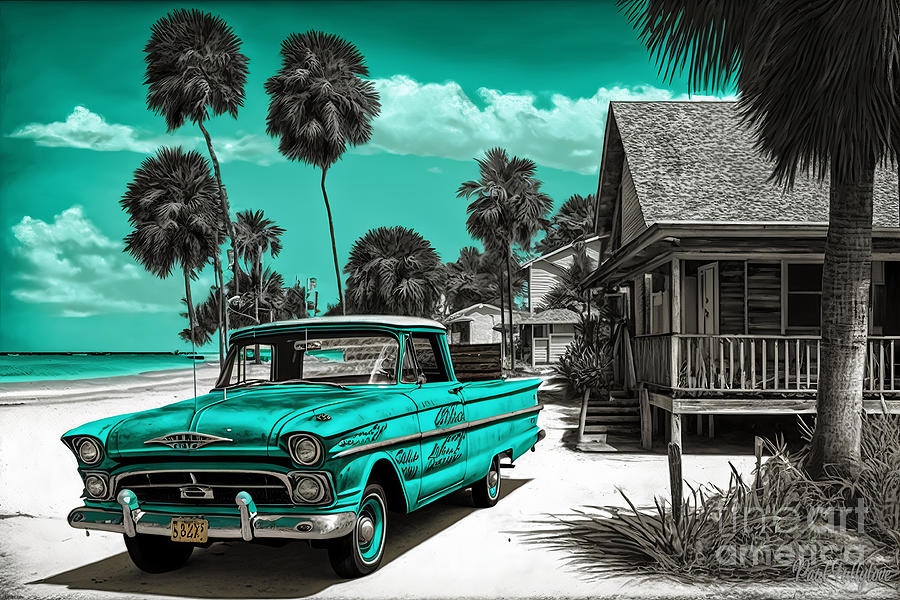This image is an illustration of a beachside resort featuring three houses elevated on stilts right on the beachfront. The sky is a vibrant turquoise with scattered white clouds, mirroring the color of a classic, turquoise Cadillac parked prominently in the foreground on the left side. This vintage vehicle, which has a shiny windshield, features a yellow front license plate and stacked headlights, possibly indicating its classic status. It also has distinctive writing on the door and near the front. The scene includes a large body of ocean with a pier visible to the left in the background. Typical beachside elements are present, such as numerous palm trees, one of which rises along the right edge of the illustration. The colorful aspects of the artwork are limited to the sky and the Cadillac, with the rest of the image rendered in black and white, giving it a striking contrast. A watermark reading "Fine Art America" is located in the bottom right corner, indicating ownership. A faint artist’s signature is also present but challenging to decipher.